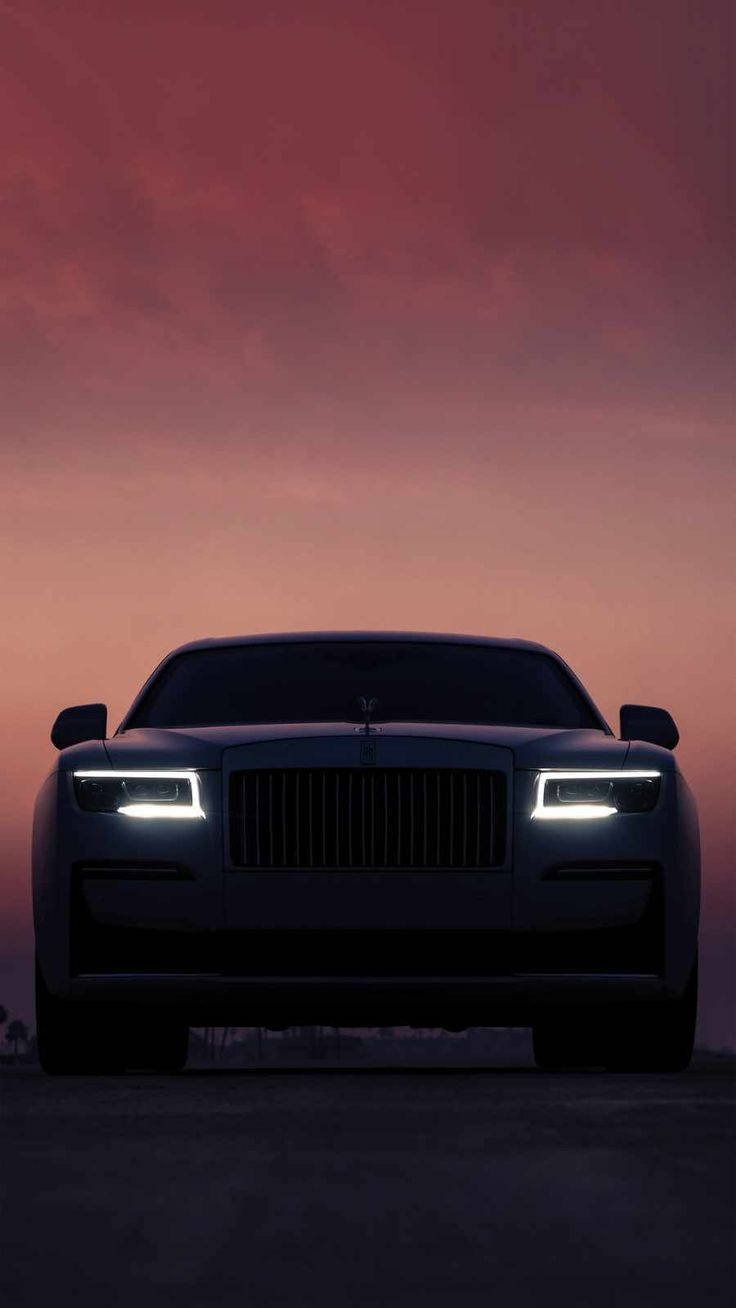The image portrays the front of a car, possibly a photo or stylized digital art, taken at dusk or nighttime. The car, enveloped in shadows, appears dark, possibly black or deep blue, with a slight purple hue, suggesting a filter may have been used. The headlights, the brightest feature, resemble stylized "U" shapes with bright white lines that create an open center. These headlights contribute a science fiction-like aura to the vehicle. The windshield and side mirrors blend into the darkness, rendering the car's interior unviewable. A subtle ornament is positioned above the middle of the large grill at the front, though its details are indistinct. The sky above is a dramatic blend of rose and purple shades, dotted with similarly colored clouds, casting a surreal backdrop. The ground beneath the car, resembling asphalt, merges with the car’s dark tones. The scene is tightly cropped, with no visible surroundings, except for faint silhouettes of palm trees against the rose-colored sky, enhancing the mystical and somewhat otherworldly atmosphere of the image.